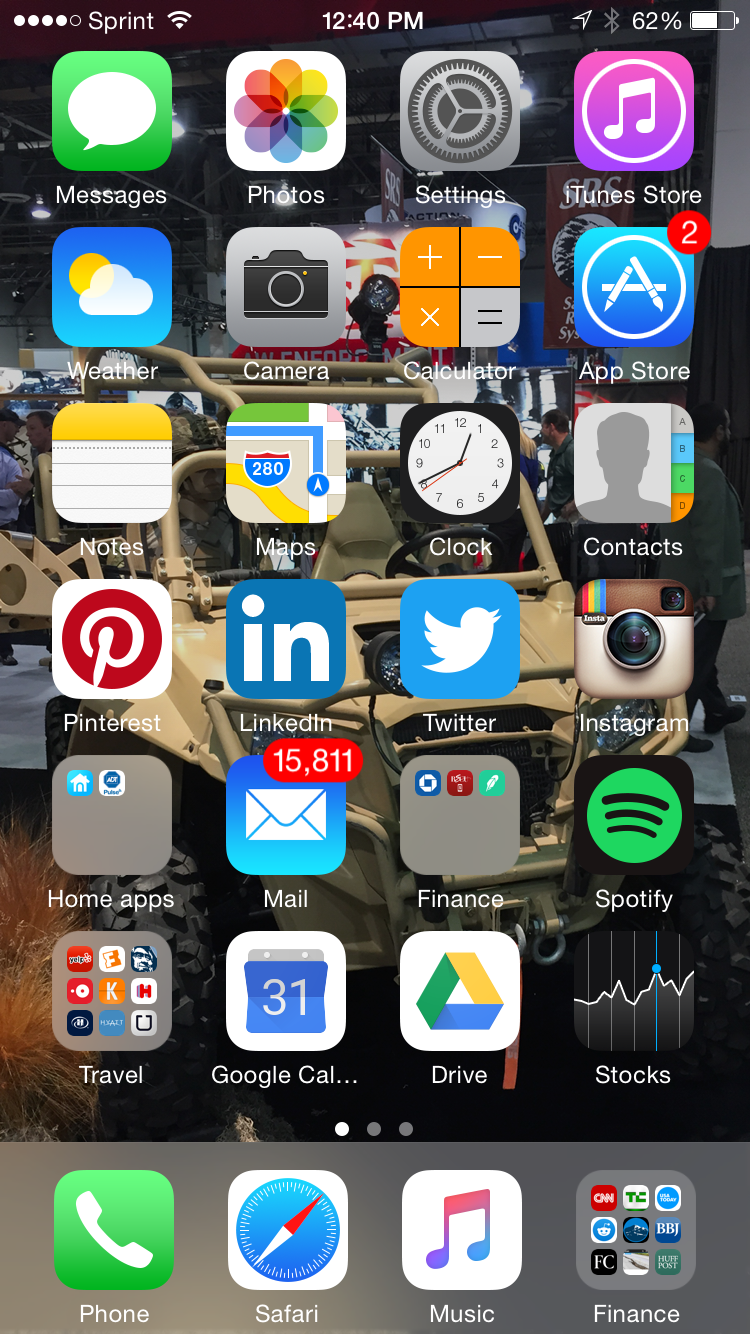This image portrays the home screen of a smartphone, specifically captured at 12:40 p.m., as indicated by the time displayed at the top. The battery status shows 62% remaining. The cellular network is Sprint, with signal strength visible in the upper left corner. Various app icons are neatly aligned across the screen. The primary row includes frequently used apps such as Messages, Photos, Settings, and iTunes. The Weather, Camera, Calculator, and App Store icons follow, with the App Store displaying a notification badge marked with a red circle containing the number 2.

The next row showcases a collection of utilities and social media apps including Notes, Maps, Clock, Contacts, Pinterest, LinkedIn, Twitter, and Instagram. Notably, the Mail app bears a red circle with an alarming 15,811 unread messages.

Further down, additional categories such as Finance, Spotify (highlighted in green), Travel, Google Calendar, and Drive are visible alongside a distinctive icon for Google Drive, recognizable by its multicolored triangular logo. The Stocks app is also present, featuring a thumbnail graph indicating an upward trend from left to right.

At the bottom of the screen, a light gray dock holds the essential apps: Phone, Safari, Music, and a folder titled Finance that includes a collection of financial applications. Overall, the organized layout provides quick access to a wide range of functionalities and services directly from the home screen.